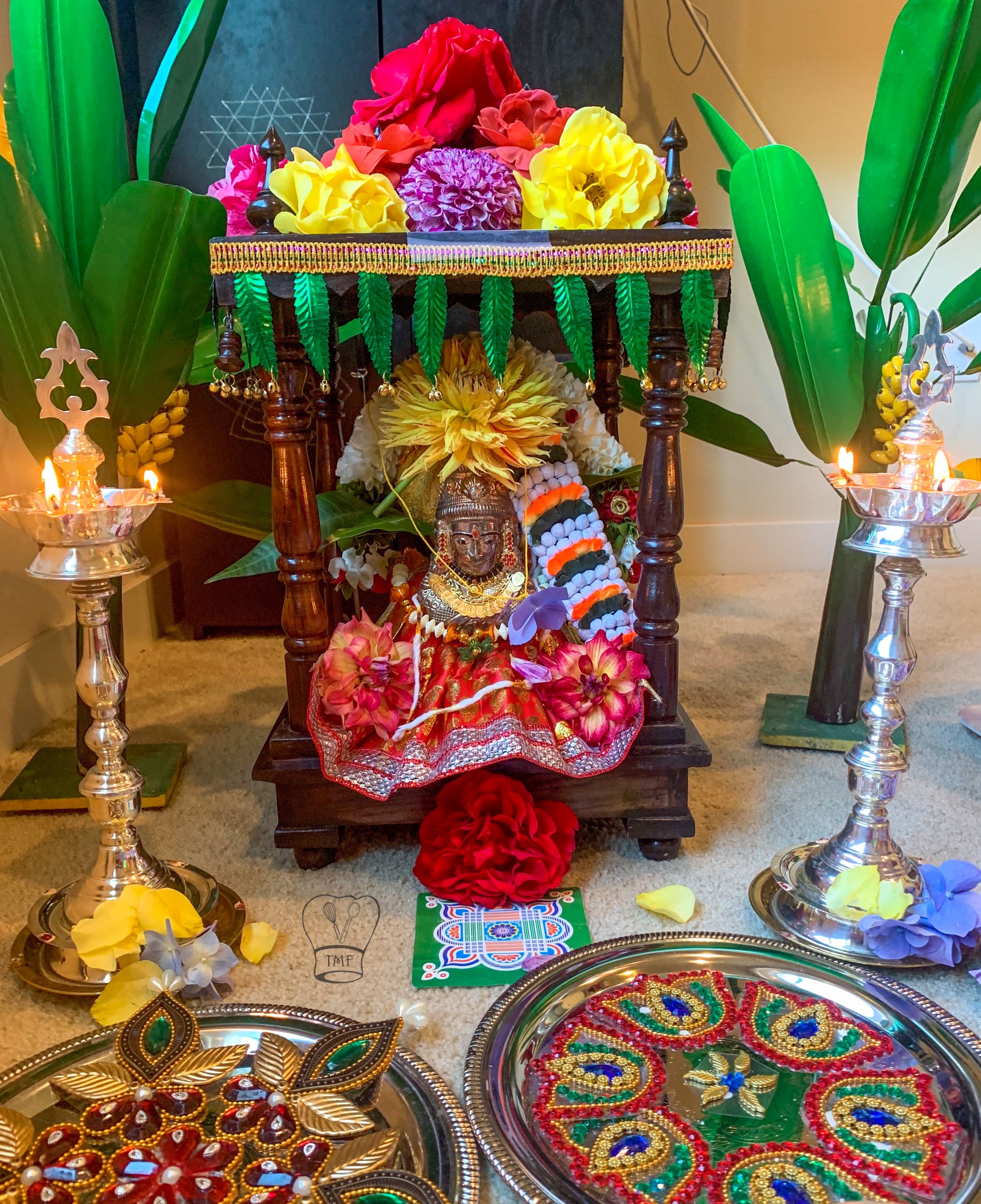The image depicts an ornate religious altar, likely within someone's home, adorned with intricate decorations and offerings. The centerpiece of the altar is a gold statue of a deity resembling Buddha, which is situated on a brown wooden table. The table is lavishly decorated with a banner featuring leaves, as well as an array of vibrant flowers including yellow, purple, and red varieties. Beneath the statue, the table is draped with a red skirt adorned with more red flowers and a mandala. The deity's head is crowned with a yellow flower, and it appears to be wearing a helmet.

Flanking the statue are two silver candlesticks with yellow petals at their bases, each holding a lit candle. In front of the altar, there are two silver platters, artistically arranged with jeweled decorations in patterns that resemble mandalas. These platters hold green, gold, and red jewels as well as pearls, adding to the opulence of the scene.

The setup is completed with additional decorative elements, including plants, flowers, and lit lanterns around the altar. The entire arrangement rests on a carpeted surface, reinforcing the impression that this reverent setup is indeed within a household environment. The photo also bears a watermark of a chef's hat with two spoons and the acronym "TMF" in the middle, suggesting the image may have origin from a specific creator or brand.